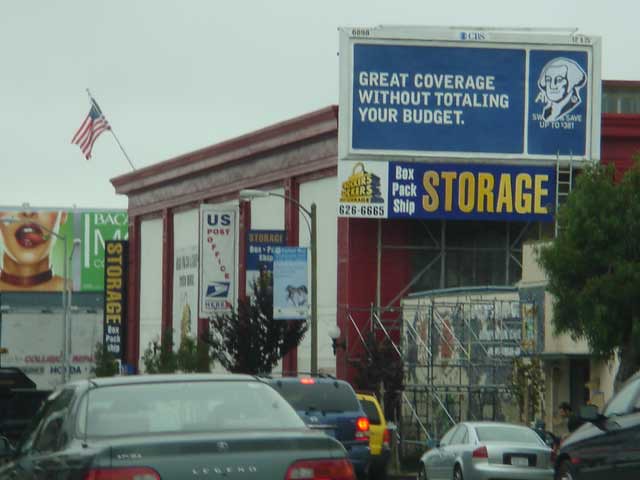In this vibrant street scene, the viewer is presented with a bustling urban landscape. The foreground is dominated by the rear ends of several cars, with a notable gray vehicle proudly bearing the "Legend" badge, alongside a dark blue car. A yellow, a silver, and a black car are also partially visible. One car has its rear lights illuminated, indicating its presence amidst the busy street.

Ahead of the cars, a prominent billboard catches the eye, featuring the lower face and neck of a woman. Adjacent to this, a black section of the billboard displays partial white text. Further to the right, a striking red building stands tall, adorned with an American flag fluttering in the breeze. The overcast gray sky adds a moody backdrop to the scene.

In front of the red building, a white sign with a blue background advertises, "Great Coverage Without Totaling Your Budget," accompanied by an image of George Washington on the left. Below this, another sign offers multiple services: "Storage, Box, Pack, Ship." Beneath these signs, scaffolding structures imply ongoing construction or renovation work on the building, contributing to the dynamic and ever-evolving urban environment.